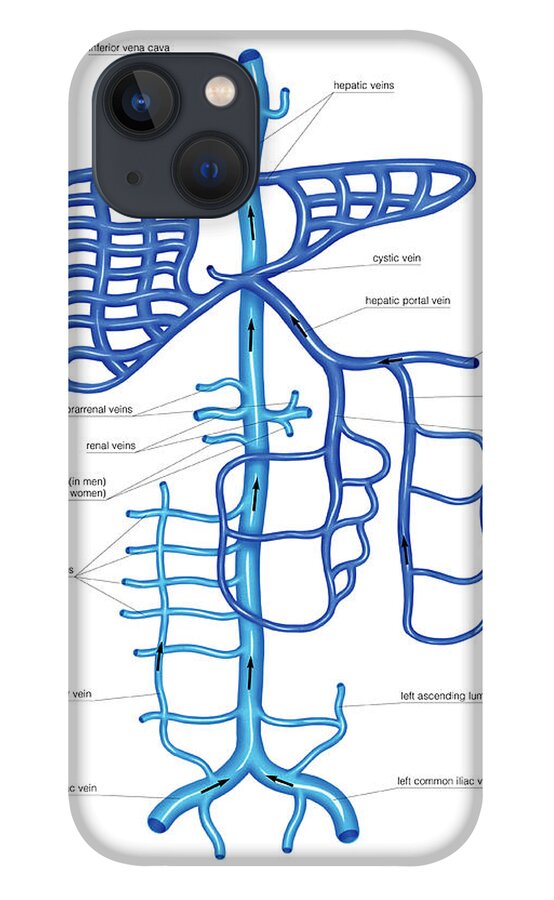This image showcases a white iPhone case with an intricate and scientifically themed design on its back. The design features a detailed diagram of human veins, rendered in various shades of blue, illustrating and labelling different components of the circulatory system. The veins depicted include the inferior vena cava, hepatic veins, cystic vein, hepatic portal vein, renal veins, and left common iliac vein, among others. Some veins are marked with arrows indicating the direction of blood flow, emphasizing the educational and anatomical nature of the design. This unique case, which likely appeals to science enthusiasts, serves as an intriguing conversation starter, given its unusual and informative appearance.